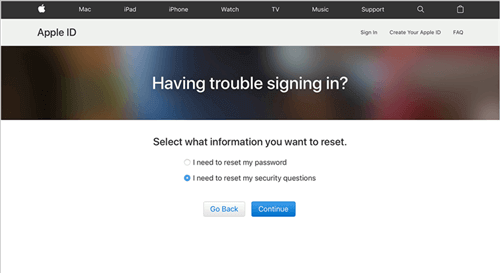Screenshot of the Apple ID Sign-In Page:

At the very top of the screen, there's a black menu bar featuring, from left to right, the Apple icon, followed by menu options for Mac, iPad, iPhone, Watch, TV, Music, Support, a search icon, and possibly a battery power icon, though it is not clearly visible. Below this, a white navigation bar displays "Apple ID" on the left, with links to "Sign In," "Create Your Apple ID," and "FAQ" on the right.

Centered on the page is a wider title bar with a dark, distorted color scheme, prominently featuring the text "Having trouble signing in?" in white lettering. The main section of the page has a clean, white background, asking the user to "Select what information you want to reset." 

Two radio button options are provided:

1. "I need to reset my password."
2. "I need to reset my security questions," with this option being pre-selected.

Below these choices are two buttons: a white "Go Back" button with blue lettering on the left and a blue "Continue" button with white lettering on the right. 

The remainder of the page is blank, focusing attention on these options and buttons. This concise layout suggests it is likely part of the Apple ID login process.